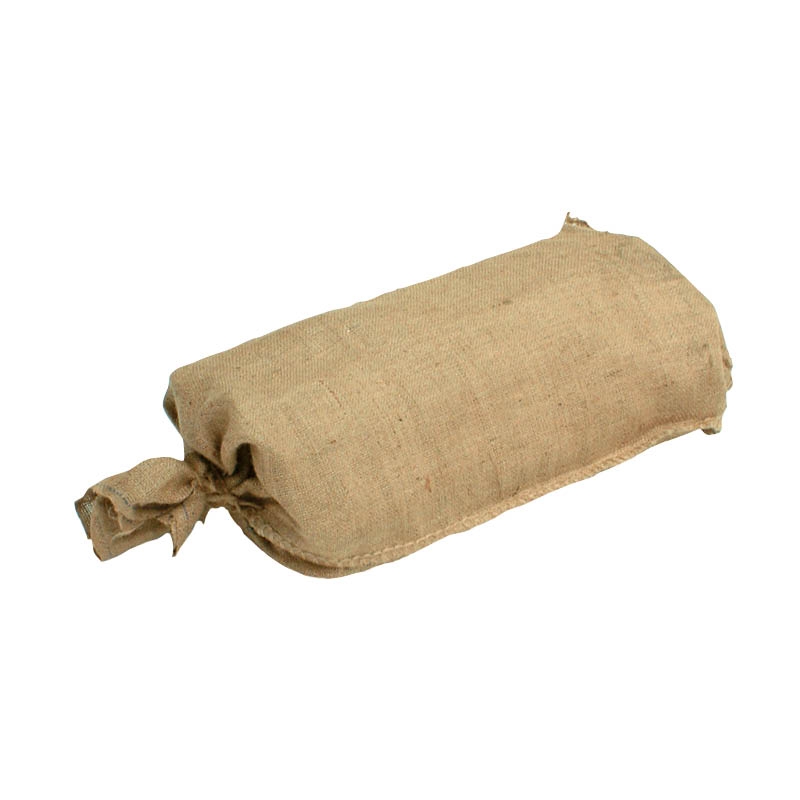In the image, a single, large brown burlap sack is prominently displayed at a diagonal angle in the center. The sack, made of a coarse, tan canvas material, is laid on its side against a completely white background, appearing as though floating in an almost blank or transparent space. The left end of the sack is bunched up and tied with a piece of braided rope that matches the color of the bag. Though it isn't completely overfilled, the sack appears to contain something that gives it a somewhat full appearance. There is also a faint hint of a blue line near the tied section. This detailed and texture-rich composition, free of any text, seems suitable for use in presentations or websites.